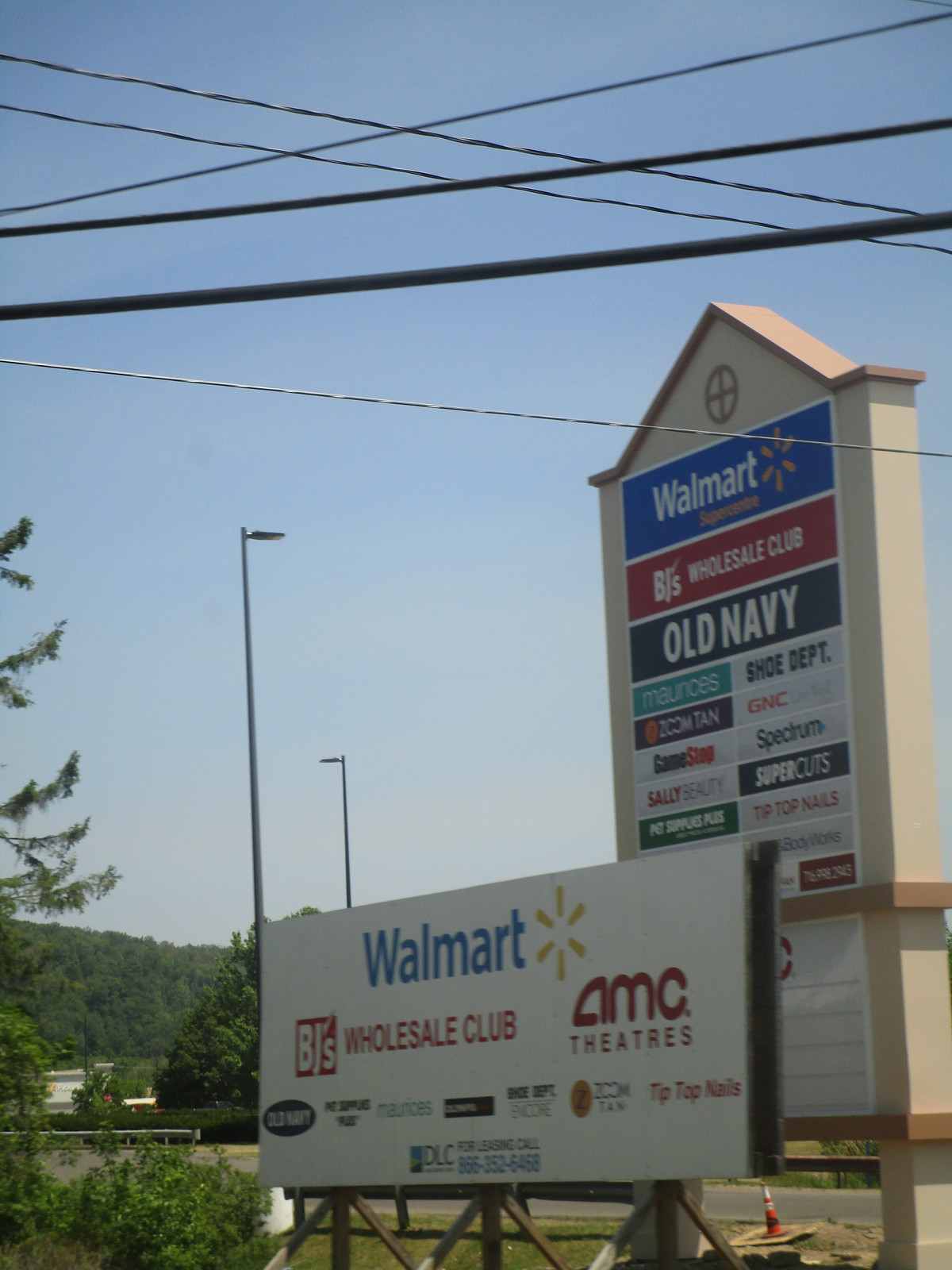The image features a vibrant blue sky with lush trees and distant mountains serving as a picturesque background for a couple of signs showcasing various retail storefronts. 

In the foreground, there is a long, horizontal billboard set against a white background. It prominently displays the "Walmart" logo accompanied by its signature yellow sunburst. Following this, the sign lists "BJ's Wholesale Club" and "AMC Theaters" in bold red lettering. Additional businesses include "Old Navy" and "Maurice's," although some of the text in between is unreadable. "Tip-Top Nails" and a phone number are also mentioned towards the bottom.

To the right of this billboard stands a taller, narrower sign that resembles a small enclosure with a peaked roof, adding some architectural depth. The topmost section of this sign features "Walmart" in white lettering set against a blue background. Descending down, "BJ's Wholesale Club" is displayed on a red background, followed by "Old Navy," possibly with a black background. Next are "Maurice's" and another unreadable store name. Further down are "Shoe Department" paired with something from "GNC," and to the left, "GameStop" and "Sally Beauty." Other stores listed include "Spectrum," "Super Cuts" (possibly misspelled as “Super Cups Cuts”), and "Pet Supplies Plus" to the left, with "Tip-Top Nails" positioned to the right. The finer details become indiscernible as the viewer’s focus continues downward.

The image captures the bustling variety of retail options available, set against the serene natural beauty of the surrounding landscape.